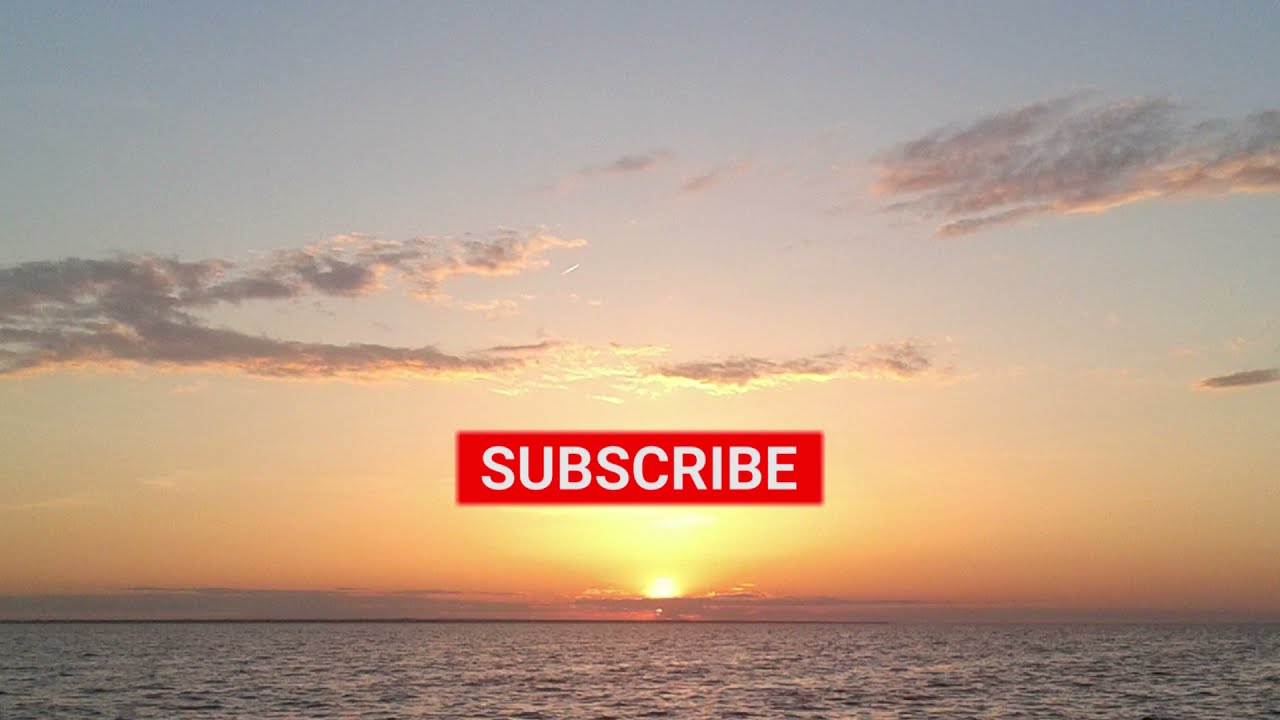The image captures a serene sunset over a vast body of water, likely an ocean or a sea. The upper portion of the sun emits a bright yellow light, transitioning to a deep orange as it nears the horizon, surrounded by a cluster of clouds. In the sky, three distinct strips of clouds are visible: the left and right ones appear larger and grayer, while the middle strip is smaller with its lower part tinged yellow by the sunlight. The expansive water below reflects an array of orange and blue hues, characterized by gentle ripples rather than waves. The overall scene is bathed in a rich palette ranging from yellow and orange near the sun to a soft pink and eventually blue in the upper sky, dotted with additional clouds that darken towards the edges. Just below the center, a red bar with the word "SUBSCRIBE" in capitalized white text suggests the image might be sourced from a video.